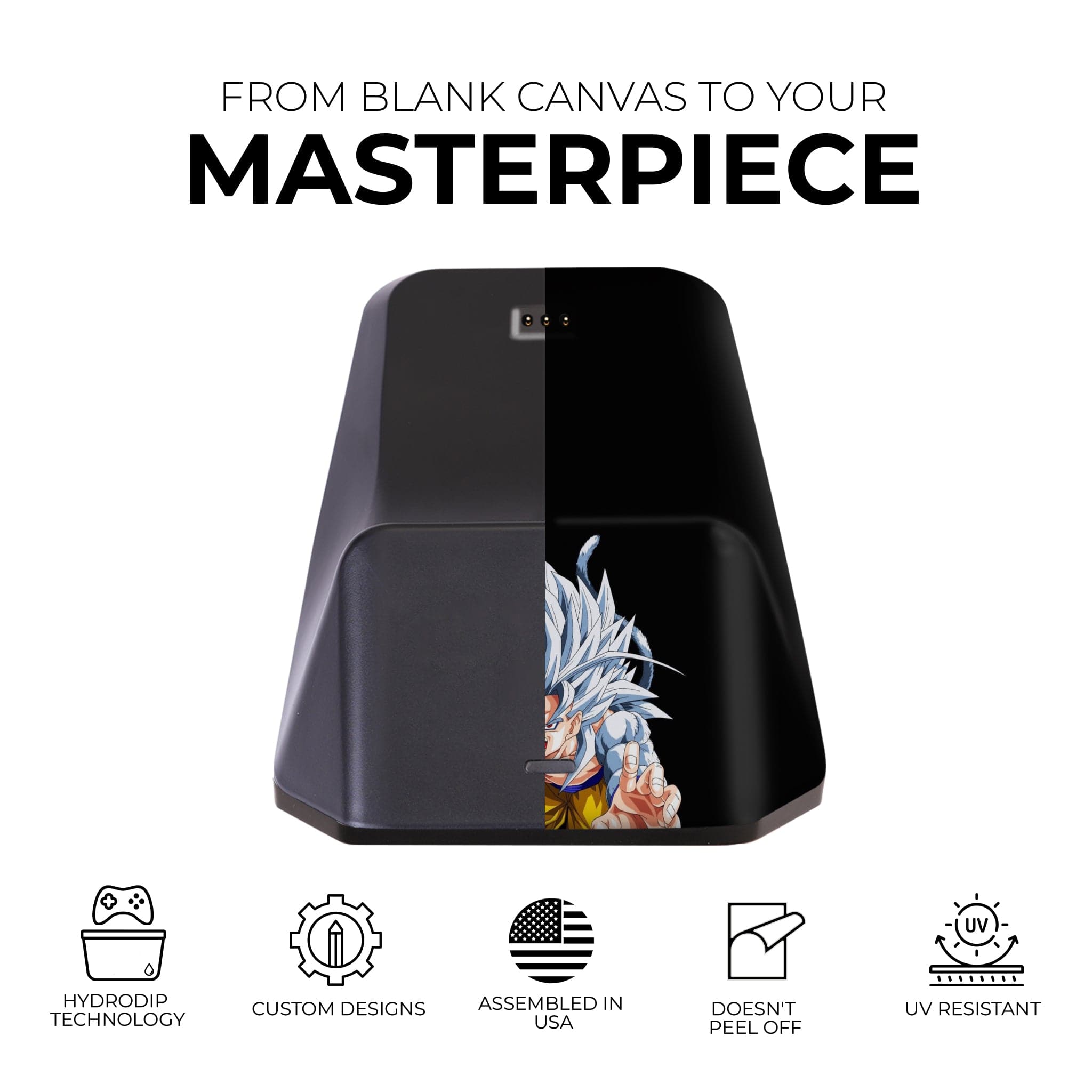The image is an advertisement featuring a customization service, possibly centered around gaming accessories or tech devices. The top of the ad prominently displays the text "FROM BLANK CANVAS TO YOUR MASTERPIECE" in bold capital letters. The focal point is a rectangular, matte black object on the left that transitions to a glossier finish on the right. The object appears to have a cover, with the center showcasing three small, mirrored spheres. Emerging from this object is a half-visible figure resembling Goku from Dragon Ball, notable for his spiky bluish-gray hair and a dynamic pose with one hand outstretched in a claw-like formation. Only half of his face is visible due to the covering.

Below this image, there is a game controller accompanied by a series of icons and text that reads: "Hydro Dip Technology, Custom Designs, Assembled in USA, Doesn’t Peel Off, UV-Resistant." Each feature has a corresponding icon, such as an American flag for the assembly location. The overall ad suggests advanced customization options for tech devices or gaming accessories, highlighting durability and unique design technology.